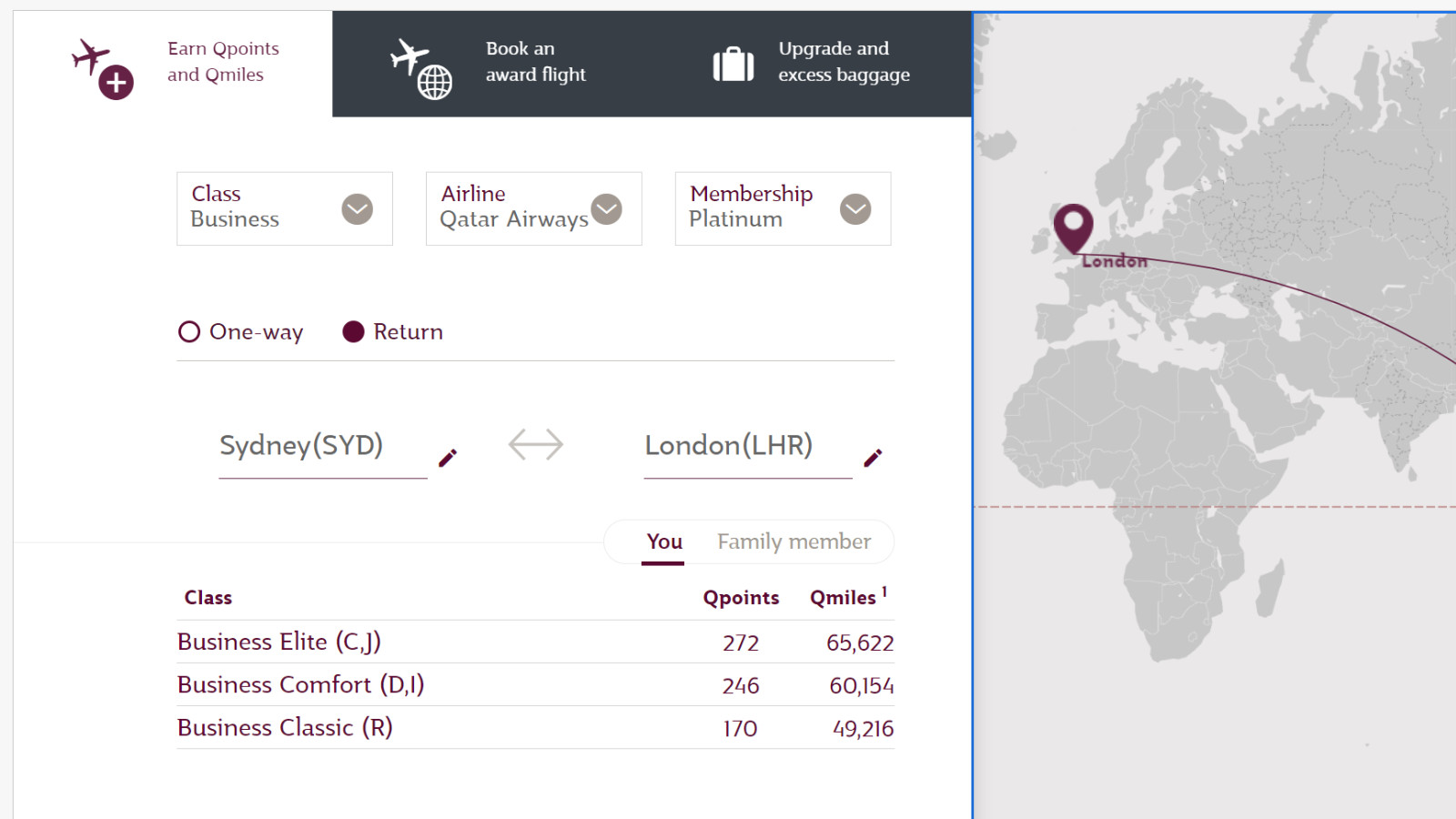This screenshot showcases detailed flight information and various travel options. The top left corner features a section labeled "Earn Q points and Q miles," marked by an airplane icon and a plus sign within a solid circle. Adjacent to this section, an airplane and Earth icon indicate the option to "Book an award flight." Following that, a suitcase icon signifies the choice to "Upgrade excess baggage." All text in these sections is written in white on a black background.

Directly below these options are three buttons. The button labeled "Class" is highlighted in red, while the "Business" option is presented in gray. Next to these is a drop-down menu indicated by an airplane icon for selecting the airline. It shows "Qatar Airways" with an airplane down arrow for additional options. Another drop-down menu labeled "Membership" displays "Platinum" with a similar airplane down arrow for further selection. Additionally, there are options to choose either "One way" or "Return," separated by a gray line.

The primary flight information given is from "Sydney to London," which can be edited via a small icon. Below this, the screen lists categories such as "Elite," "Comfort," and "Classic," alongside options for "Family members" to accumulate "Q points" and "Q miles." On the right-hand side, there’s a graphic showing a map with continents, specifically highlighting Africa and Europe, and pinpointing London as a destination.